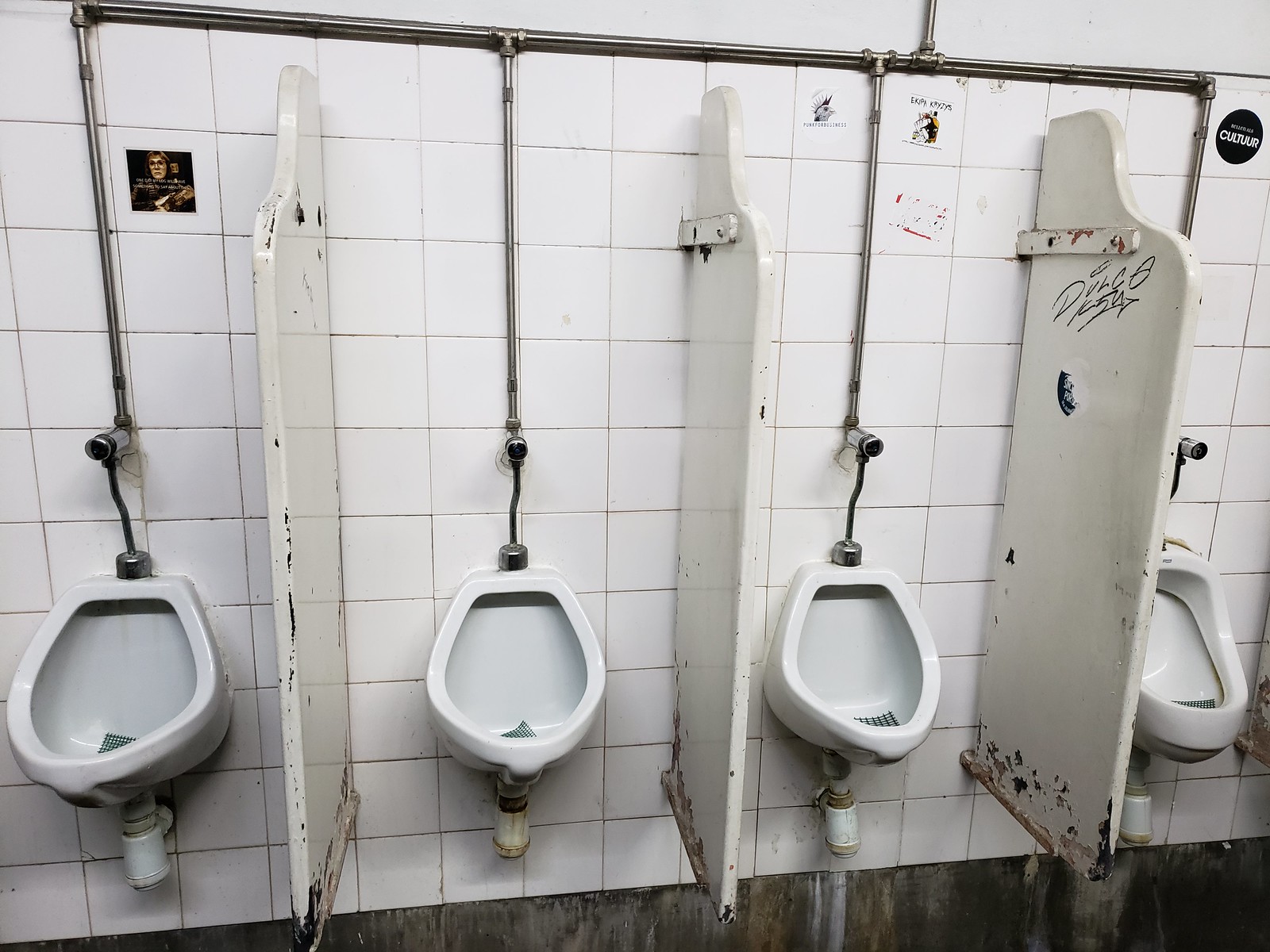This photograph depicts an old, unclean men's public restroom featuring four white urinals mounted against a wall of large, square white tiles. Each urinal is separated by a thin, white divider that shows noticeable wear, with chipping paint and graffiti. Above the urinals, a series of silver pipes run horizontally along the top of the image, with perpendicular pipes extending down to each urinal. The floor is barely visible but appears shiny and possibly reflective. The restroom ambiance is further marred by several stickers and pieces of graffiti: a black and white picture on the tile above the first urinal, three small stickers in the third stall, and a circular black sticker bearing the word "culture" in the final stall. The overall appearance of the bathroom is outdated and neglected, adding to its unsanitary impression.